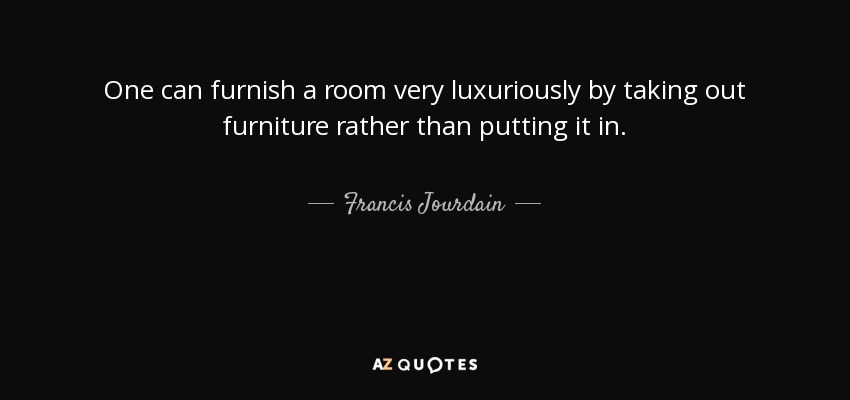The image features a solid black rectangle with centered white text. At the top, in a serious and professional font, it reads: "One can furnish a room very luxuriously by taking out furniture rather than putting it in." Beneath this quote, the author's name, "Frances Jourdain," is displayed between two long hyphens in a playful, cursive font. At the bottom of the image, "AZ QUOTES" is centered, with the letter "O" in "QUOTES" replaced by a speech bubble icon, which is white with black filling. Additionally, the letter "Z" in "AZ" is highlighted in a peach color, contrasting with the otherwise white text. There are no other images or icons, just the text centered throughout the black rectangle.